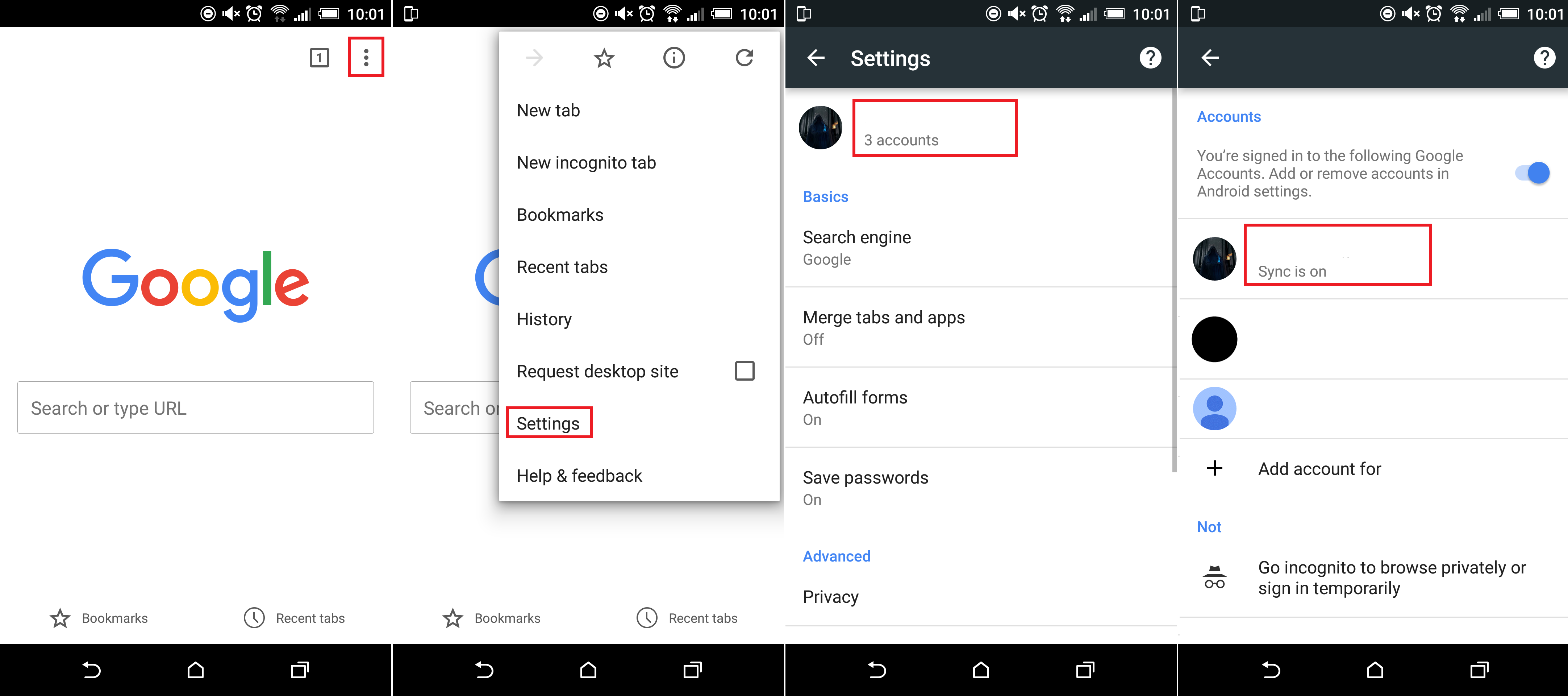The image depicts a step-by-step guide on how to navigate certain features in the Google Chrome browser. The interface shows multiple tabs open, with the primary tab displaying Google's homepage, which includes the familiar search bar in the center of a blank screen.

A red square highlights the three vertical dots in the upper right-hand corner, indicating the menu icon and the first step in the tutorial. Adjacent to this, another screen shows the expanded menu with the 'Settings' option encircled, emphasizing it as the next action.

The following screen, positioned side-by-side, displays the 'Settings' page, listing options such as 'Basics', 'Search Engine', 'Merge Tabs and Apps', 'Autofill Forms', 'Save Passwords', and 'Advanced Privacy.' Under the 'Accounts' section, it shows that users are signed into a Google account, with instructions to 'Add or remove accounts in Android settings.' The guide specifies that the first account is highlighted and notes that 'Sync is on.'